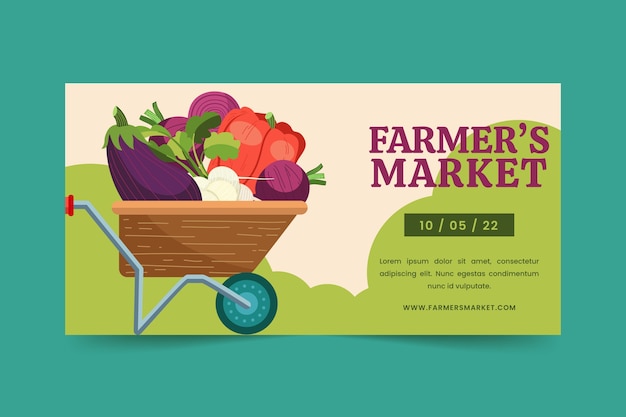The image serves as a detailed advertisement for a farmer's market, styled in a cartoonish digital drawing format that could be the size of a business card. The overall layout features a teal border, accentuating an off-white upper section and a green lower section. Dominating the left side of the image is a brown wheelbarrow with a distinctive wood grain pattern. The wheelbarrow includes a red handle, a steel frame, and a cyan-colored wheel, adding a playful, multicolored aesthetic. 

The interior of the wheelbarrow is filled to the brim with oversized vegetables—eggplants, onions, red bell peppers, and purple radishes—carefully illustrated to grab attention. These vegetables rest in a basket that sits atop a metal base, combining rustic charm with industrial sturdiness. Surrounding the wheelbarrow, the backdrop features a combination of beige and green hues, with green areas designed to resemble bushes or hills, enhancing the agricultural theme.

Adjacent to this scene, on the right side of the image, is the event information. "Farmer's Market" is prominently displayed in bold purple text. Below that, a dark green rectangle contains the date "10-05-22" in light green text, signaling the event's occurrence. Further down, there is placeholder text in Latin, followed by the URL "www.farmersmarket.com," all in green text, providing additional details and a point of contact for interested attendees.